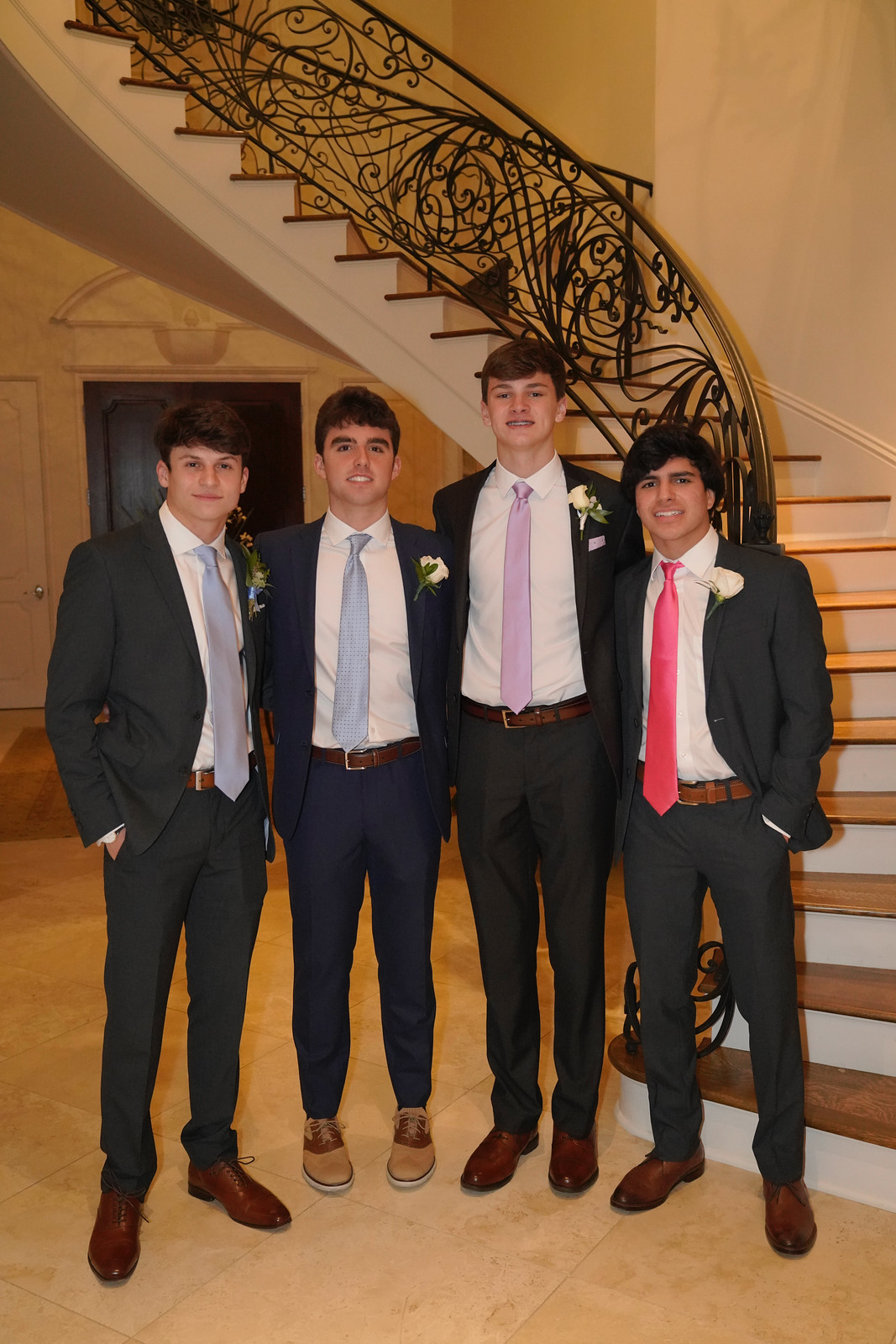The photograph depicts four young men, likely in their late teens to early twenties, dressed in well-fitted suits, standing together indoors in front of a striking spiral staircase. Each of them is clad in single-breasted suits with trouser slacks featuring a seam down the legs, complemented by white shirts, ties, and brown belts. Notably, the first, third, and fourth men wear black suits, while the second man differentiates himself in a dark blue suit.

Their ties add a splash of color to their attire: the first man sports a powder blue/periwinkle tie, the second a slightly darker pale blue tie, the third a lavender tie, and the fourth a carmine red tie. Each of them has a flower pinned to their lapel, suggesting they might be part of a wedding party or attending a formal occasion.

The young men all wear brown dress shoes, although the second man from the left stands out with his tan leather shoes that lack the shiny finish seen on the others' shoes. They all have brown hair and tan skin, and the third man appears to be wearing braces, giving further indication of their youthful age.

The setting features a grand spiral staircase with ornate black wrought iron railings adorned with intricate curves and curls, topped with what appears to be a copper finish. The staircase itself has wooden steps with white vertical risers. The floor beneath them is described as ceramic or marble, adding to the elegance of the scene. The lighting in the photo includes a slight flash effect, enhancing the clarity and prominence of the subjects against the sophisticated backdrop.